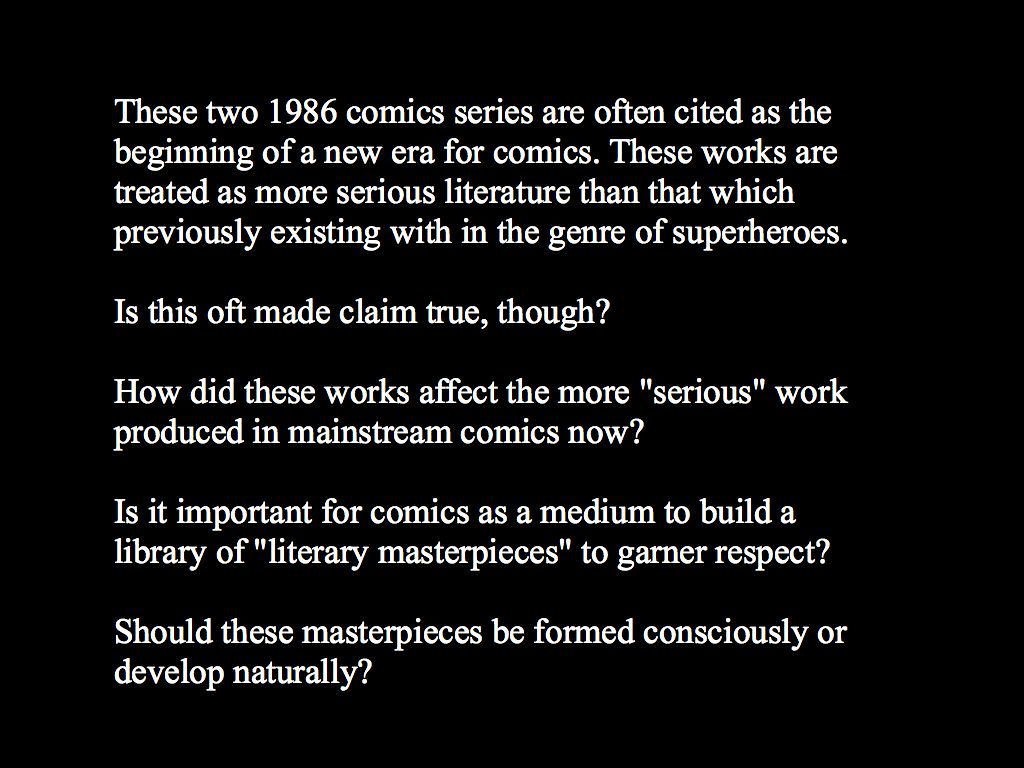The image consists of a solid black rectangular background filled with white text. The text reads: "These two 1986 comic series are often cited as the beginning of a new era for comics. These works are treated as more serious literature than that which previously existed within the genre of superheroes. Is this oft-made claim true, though? How did these works affect the more serious work produced in mainstream comics now? Is it important for comics as a medium to build a library of literary masterpieces to garner respect? Should these masterpieces be formed consciously or developed naturally?"